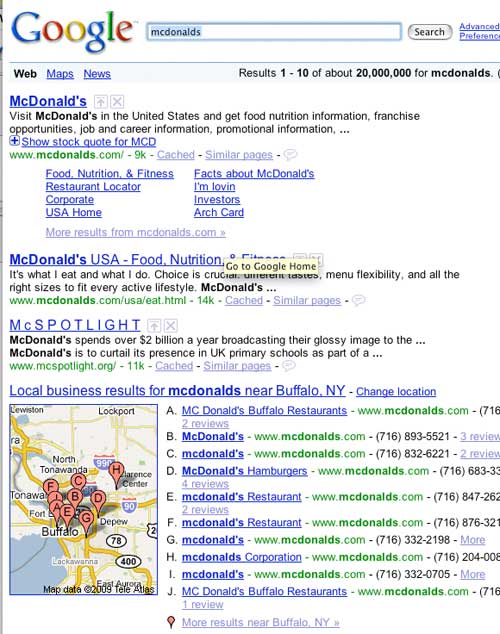The image is a detailed screenshot of an old Google search page from around 2009, indicated by a "map data, circa 2009, TeleAtlas" note on the map at the bottom of the webpage. At the top, the classic Google logo is displayed with its vintage, thin, and colorful design: a blue capital 'G', followed by a red 'O', a yellow 'O', a blue 'G', a green 'L', and a red 'E'. To the right of the logo is the familiar search bar, containing the term "mcdonalds" in lowercase without an apostrophe. The search term and the search bar are highlighted in blue, suggesting it is active or selected by a mouse.

Adjacent to the search bar is a rounded, metallic-button search icon, reminiscent of the old Apple OS aesthetics. To the right of this, hyperlinked text reads "Advanced Preferences". Below the search bar is the Google navigation bar, featuring buttons for "Web", "Maps", and "News". The "Web" option is selected, appearing bold and black, while "Maps" and "News" are blue and underlined.

The search results indicate entries "1 to 10 of about 20,000,000 for mcdonalds". The top search result links to the official McDonald's website, followed by a link to the McDonald's USA food and nutrition information. The third link points to "McSpotlight". Additionally, there are localized business results for McDonald's locations near Buffalo, New York, displayed via a map populated with pins denoting each location.